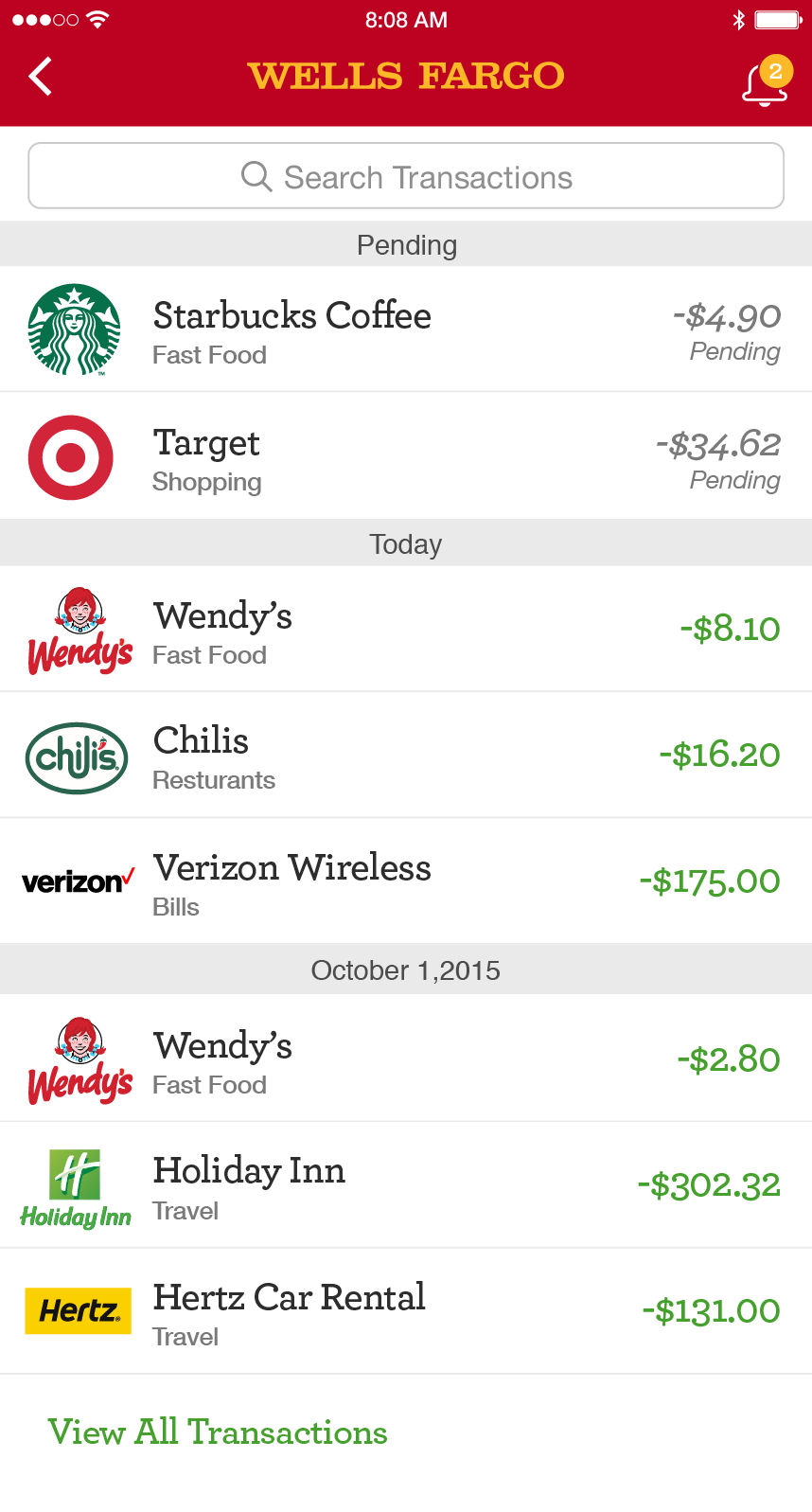The image is a screenshot of a mobile banking app interface with a detailed transaction history. The background is brown, and at the top of the screen, the device shows icons indicating cell phone signal strength, Wi-Fi strength, the current time (8:08 AM), Bluetooth status, and a full battery.

Underneath, the interface displays a back arrow on the left side, a yellow Wells Fargo logo, and a bell icon with the number "2" indicating notifications. There is also a search bar for transactions, with white text on a gray background.

The transaction list begins with the section labeled "Pending" (gray text on a gray background):

1. Starbucks Coffee: -$4.90 (pending)
2. Target: -$36.62 (pending)

Following the pending transactions, today's completed transactions include:

1. Wendy's Fast Food: -$8.10 (gray)
2. Chili's Restaurants: -$16.20 (green)
3. Verizon Wireless Bill: -$175.00 (green)

Further back in the transaction history:

1. October 1, 2015: Wendy's Fast Food: -$2.80 (green)
2. Holiday Inn Travel: -$302.32 (green)
3. Hertz Rental Car: -$1.31 (green)

At the bottom left of the screen, there is an option to "View Transactions" highlighted in green. 

Overall, the screenshot sums up recent and pending financial activity on the user's account.